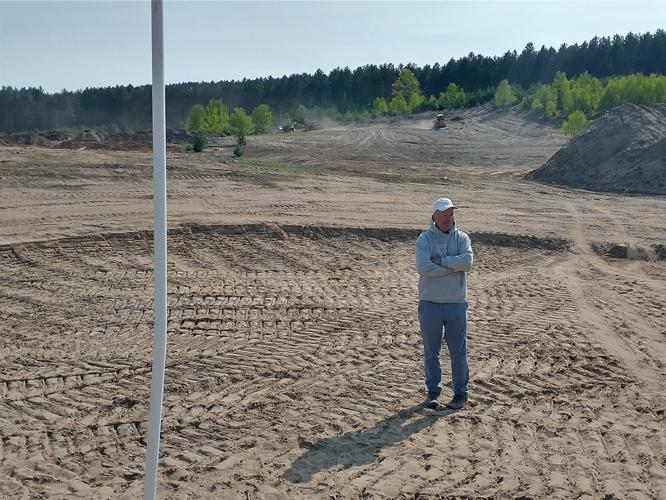This is a highly detailed color photograph capturing a man standing in the middle of a large, cleared dirt field, likely a new construction site. The ground is grayish-brown, covered in a dirt or sand-like substance, and it features numerous tire tracks forming a circular pattern around the man, possibly from large construction vehicles. The man, standing slightly off-center to the right of the image, is wearing blue jeans, a white sweatshirt or hoodie, a white baseball cap, and work boots; his arms are crossed over his chest as he looks downward. A prominent white pole is visible on the left side of the image, though it is cut off at the top and bottom, making its purpose unclear. In the background, there is a tree line indicating proximity to a forested area, along with a pile of dirt and what appear to be two pieces of heavy machinery, possibly bulldozers, partially visible near a rocky formation on the top right. This image depicts a serene yet industrious scene, highlighting the early stages of land development.